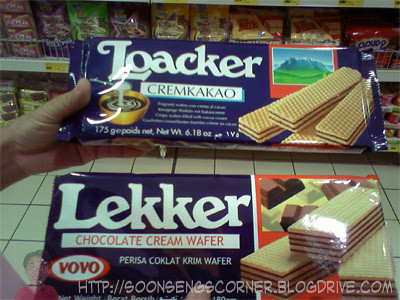The image depicts a person holding two packages of wafer cookies within what appears to be a supermarket snack aisle. The focus of the image is on the hands and the wafers they are holding, with white square tiles featuring gray grout visible on the floor. The background reveals shelves stocked with various food items. The person's left hand is holding a dark blue package labeled "Loacker Creme Cacao," featuring images of wafer cookies, cream, and a scenic backdrop of a garden and mountains. Their right hand holds another dark blue package labeled "Lecker Chocolate Cream Wafer," which also displays images of chocolate wafers and pieces of chocolate. Small textual details on the packaging include some partly visible numbers and descriptions. At the bottom corner of the image, a URL is visible: http://soosangscorner.blogdrive.com.